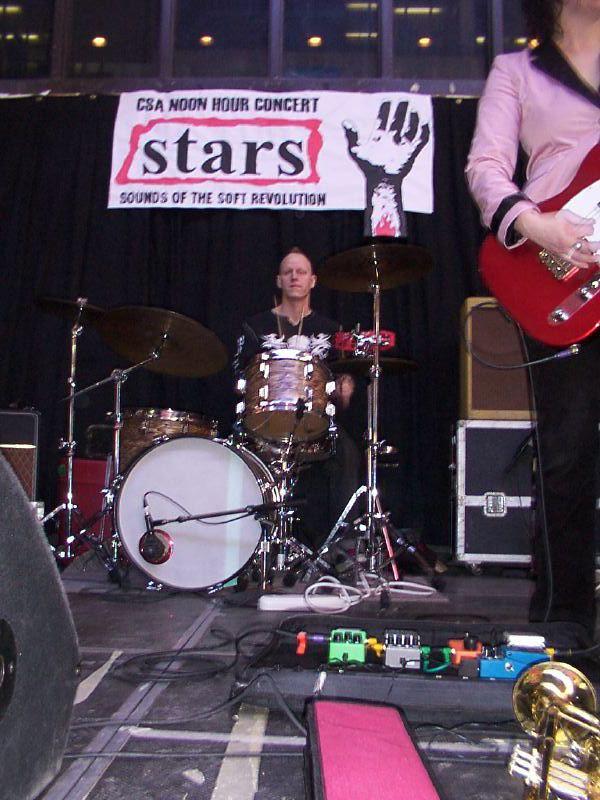The image depicts a lively concert stage, featuring a drummer with a thin, short mohawk, playing a drum set adorned with a wooden veneer around the snares. He is wearing a black t-shirt with white writing, likely a death metal logo. A young woman is partially visible to the right, playing a red guitar with white markings. Behind the drummer, a large banner reads "CSA Noon Hour Concert" with "Stars" enclosed in a red-lined border, followed by "Sounds of the Soft Revolution." A prominent black-and-white image of a hand reaching up with fingers outstretched is part of the banner. The stage is filled with various equipment boxes, a switching box, electrical connectors, and a brass-colored trumpet with silver valves slightly visible. The overall lighting suggests a possibly natural outdoor environment, but this detail is not certain.